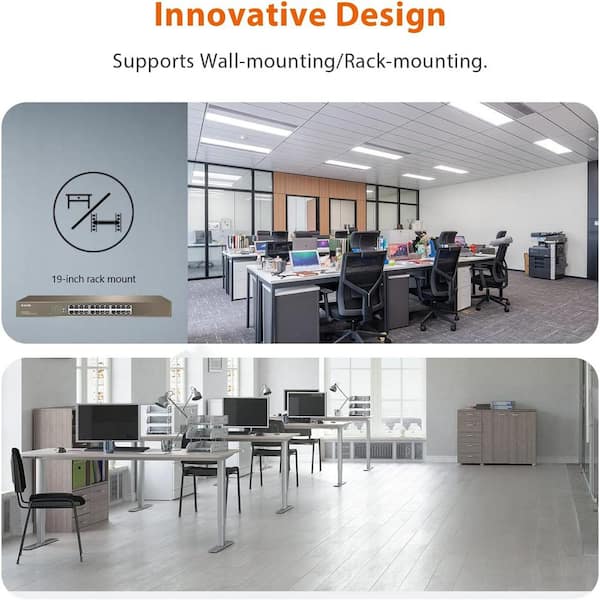The image is a before and after depiction of an office space redesign. At the very top of the picture, bold and large orange text reads "Innovative Design," followed by smaller text indicating "Supports wall mounting, rack mounting," and "19-inch rack mounting." The upper part of the image shows a photo of the 'before' state, where the desks are cluttered and crowded together in the middle of the space, with chairs lined up in front of an office table that accommodates three seats. The scene appears disorganized and cramped. Below, the 'after' photo reveals the reimagined office, featuring individual tables and a noticeably more open and organized layout. The transformation highlights a modernized and efficient workspace with a variety of colors including light brown, gray, black, purple, pink, and green.